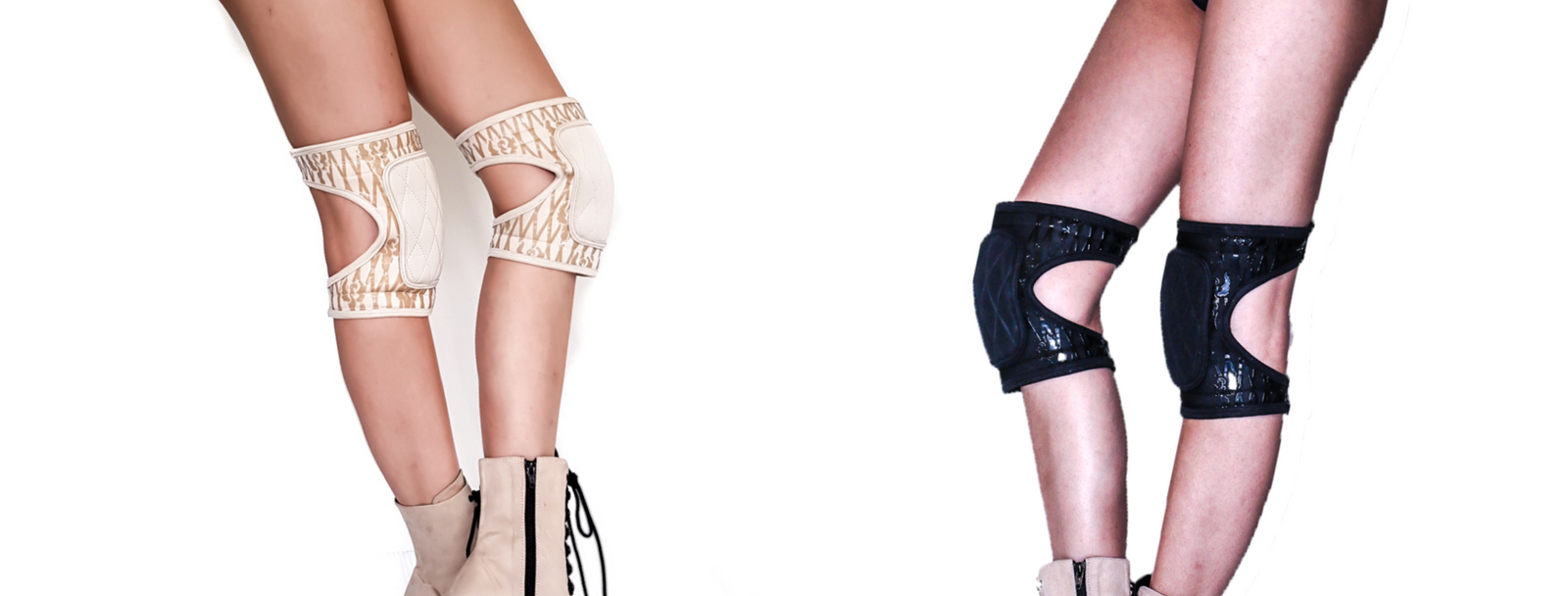The photograph showcases the legs of two fashion models against a pure white background, highlighting an aesthetic contrast in their attire and accessories. Both models, who appear to be white women, have smooth, hairless legs extending from the upper thigh to just below the knee. The model on the left has slightly more tan skin and is adorned with cream-colored knee pads that feature a vertical rectangle of padding in the front and an open back for mobility. Strapped around her knees, the pads sport light brown triangle designs. She is also wearing tan-colored roller skates with black zippers and laces, visible up to the ankle. The model on the right, with lighter skin, wears black, shiny knee pads that similarly have a vertical padded section in the front and an open back. Her attire includes cream-colored roller skates, partially visible with black detailing. Both sets of legs are positioned to face inward, creating a mirrored composition. The background's stark whiteness accentuates the minimalist and contrasting color palette of their knee pads and roller skates.